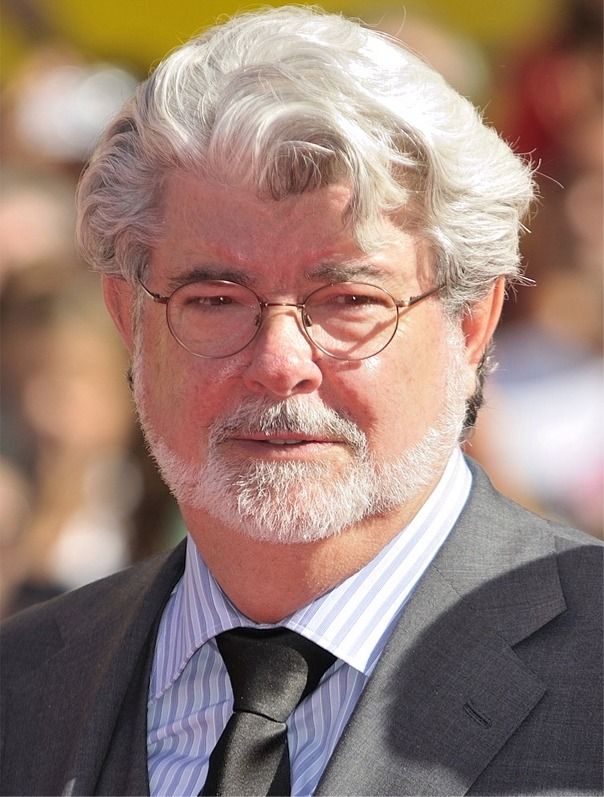This is a detailed photographic portrait of an elderly Caucasian man, who is likely in his 50s or 60s, possibly even older. Prominently featured with fluffy white hair coiffed to the side and a high brow, his head is parted left to right. He has a neatly trimmed white beard, mustache, and a goatee. His facial expression is serious, almost squinting, as he looks directly at the camera with his mouth slightly open, revealing his two front teeth. The man is distinguished by his thin wire-rimmed circular glasses and is dressed formally in a light gray suit paired with a blue and white vertically striped shirt and a matching gray tie. The background of the image is a blurred mixture of green and red hues, ensuring that the focus remains on him. There is no text within the image. Some suggest this might be George Lucas, renowned director of the Star Wars movies, although there is no confirmation.